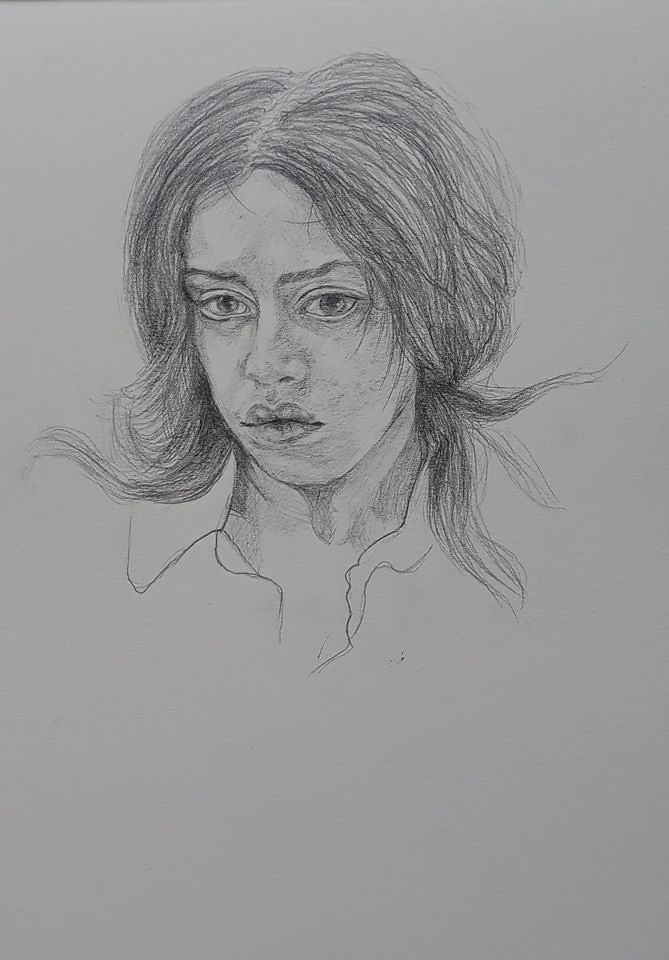This is an exceptionally detailed pencil drawing of a young girl rendered in black and white. The portrait takes up the top half of the paper, leaving a considerable amount of blank space below. The girl is looking directly at the viewer with a sulky, sad expression that suggests she's seen something distressing. Her prominent, expressive eyes appear to be brown due to the shading, and they are downcast, adding to her overall forlorn appearance.

Her eyebrows are thin and set low on her forehead, contributing to the sorrowful look. She has very full lips and a normal-sized nose. Her hair is messy and unkempt, parted down the middle and touching just above her shoulders. It seems to have been tied back neatly at some point but is now frayed and disheveled. The detailed shading around her neck gives a sense of depth and dimension to the drawing, and you can see the beginnings of a shirt collar, though most of the lower half of the paper remains blank. The artwork is intricately done, capturing the essence of the girl's melancholy with great precision.